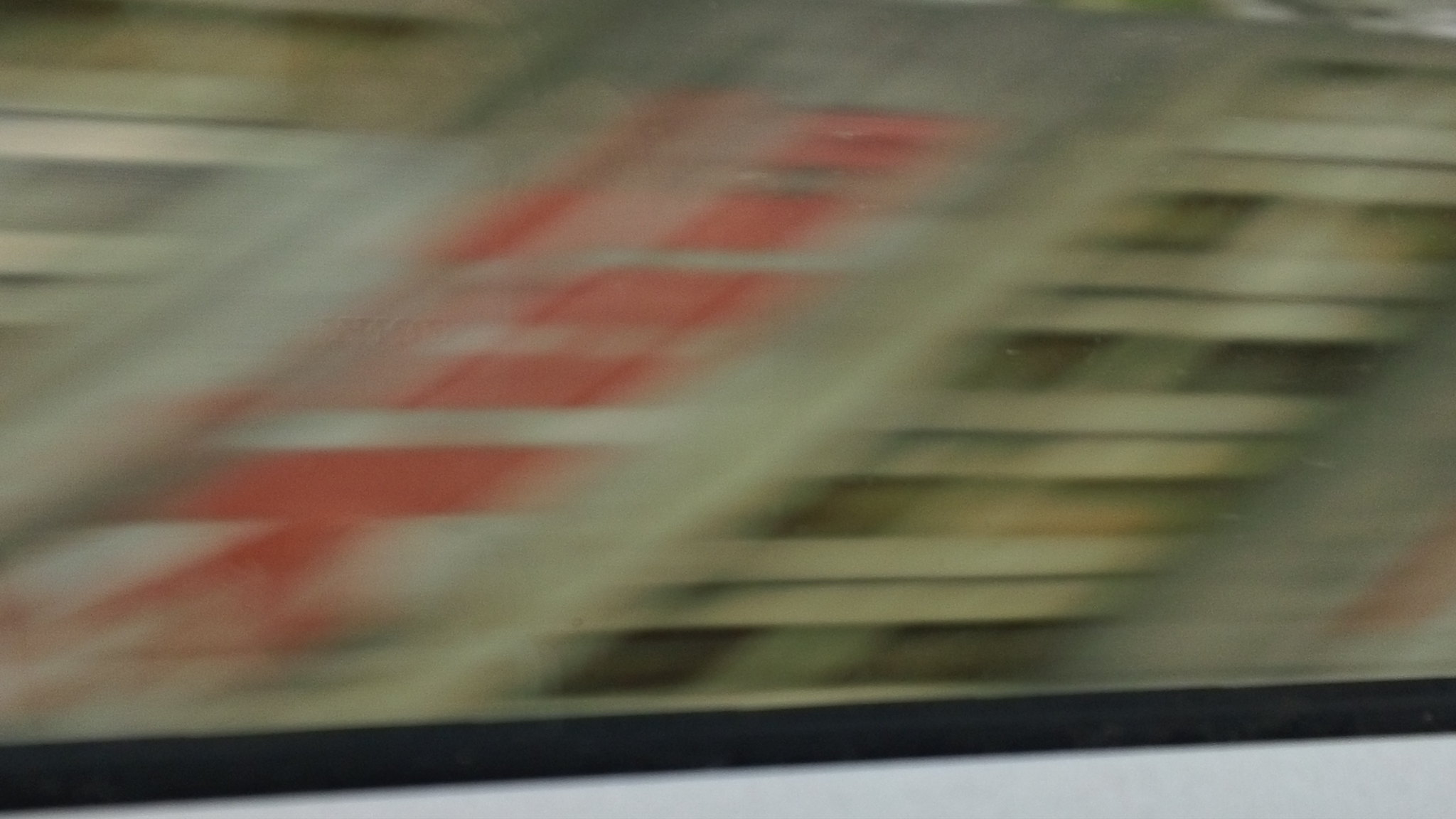The image is a blurry, somewhat indistinct photograph likely taken from a moving vehicle, possibly a car or bus, through a window with a black line at the bottom, possibly indicative of a window frame. The scene depicts an industrial setting, possibly the interior of a building or the underside of a roof, characterized by exposed wooden beams or structures that resemble slanted ladders. There are notable colors such as silver, red, and a light brown or khaki that dominate the image, contributing to an aged, off-white, and weathered appearance. Additionally, there are several diagonal elements running from the lower left to the upper center of the photo, which could be opaque or transparent structures hinting at blinds or slats, creating a layered and somewhat chaotic impression. Overall, the image blends industrial elements with the motion blur from being captured in a moving vehicle, making the exact details difficult to distinguish.